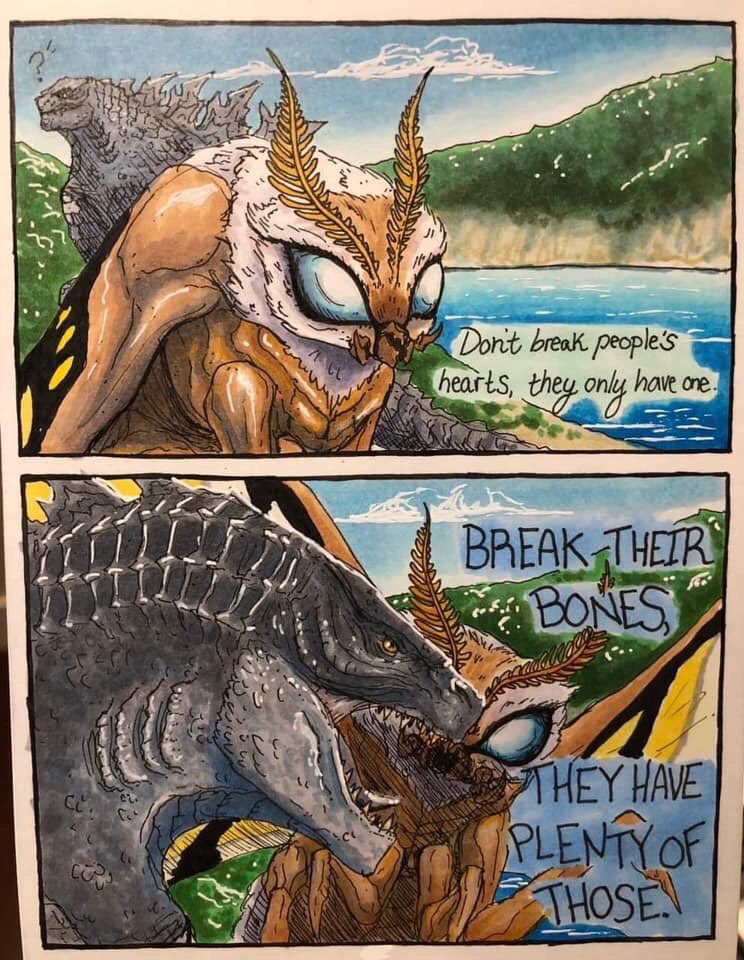This is a detailed cartoon drawing divided into two panels. The upper panel features a unique insect-like creature with feathered appendages above its nose and notably thick biceps. This creature, characterized by its brownish body and light blue eyes, stands by a lake with green and brown mountains in the background. Behind it looms a gray, Godzilla-like monster with sharp bones protruding from its back and a scaly texture. The insect is speaking, with a caption that says, "Don't break people's hearts. They only have one."

In the lower panel, the scene shifts dramatically as the aforementioned monster, now appearing more clearly like a Tyrannosaurus rex, attacks the insect. The monster has the insect's head in its mouth. This panel maintains the scenic backdrop of the green mountains. The attacking monster mockingly says, "Break their bones. They have plenty of those." The juxtaposition of the peaceful advice in the upper panel against the violent reality in the lower one adds a layer of dark humor to the comic.